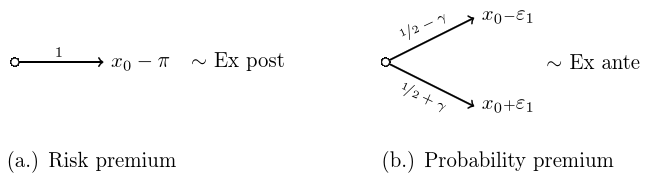In this photograph, a complex mathematical equation is being analyzed. On the left side of the image at the bottom, there is a notation "RISK PREMIUM" enclosed within two commas and a dot. Just above this, there's a circle intersected by a line with an arrow pointing upwards, labeled with the number "1". Adjacent to this, the terms "X₀ YNS" are written, followed by a small drawing of a line branching into two directions with a wavy line beside it, labeled "EX POST".

On the right side of the image, the term "PROBABILITY PREMIUM" is written next to a "B" dot. Above this term, there is a circle with two lines extending from it in opposite directions, each tipped with arrows. The top line is annotated with "½ - Y" and the bottom line with "½ + Y". Next to this diagram, there are the terms "X₀ - E₁" on top and "X₀ + E₁" below. A wavy line beside the entire diagram is marked with the notation "EX ANTE".